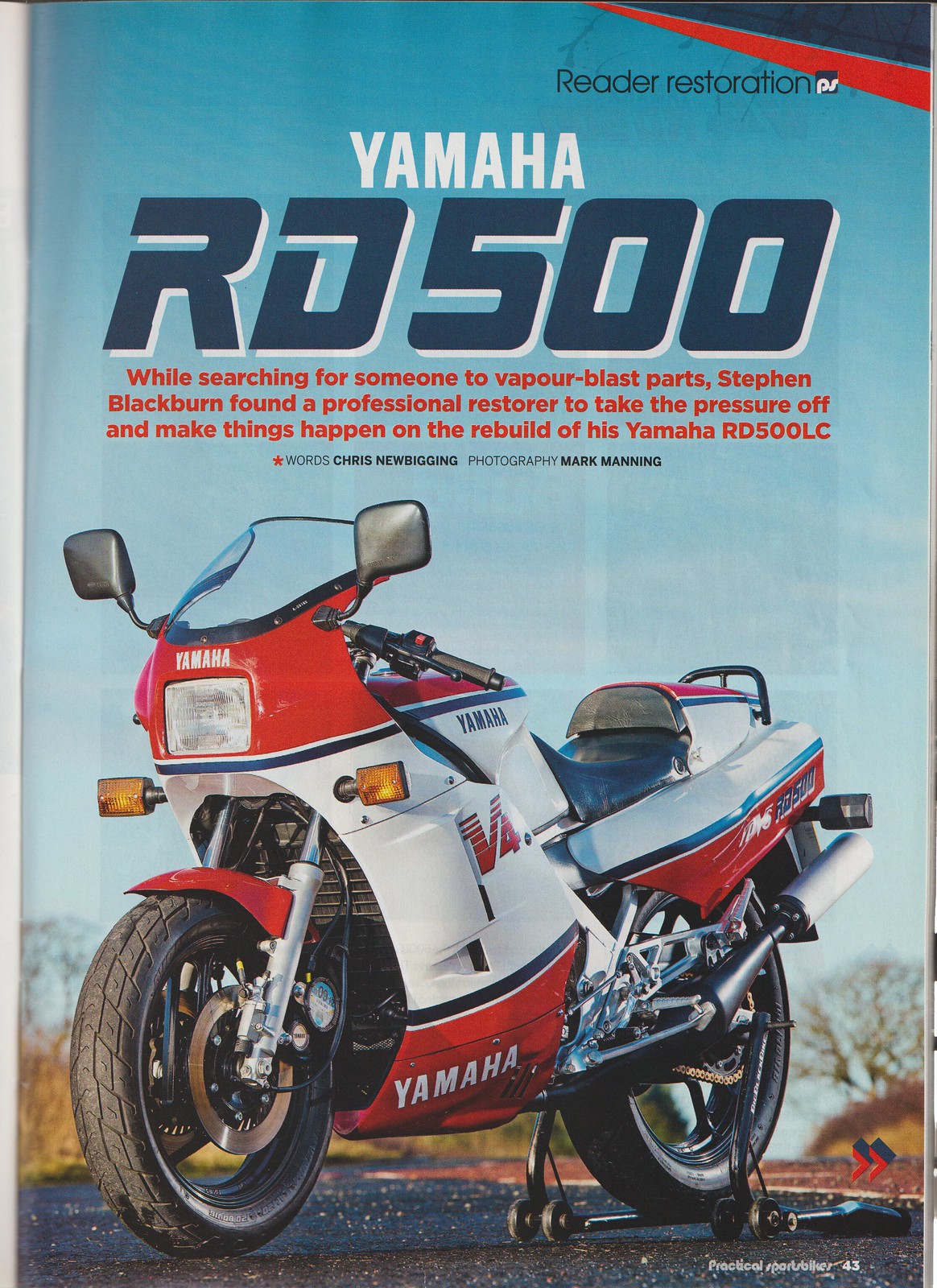The image presents a full-page magazine spread featuring the headline "Reader Restoration" prominently at the top right. In the center, large white text spells out "Yamaha RD500," with a subtext below it reading: "While searching for someone to vapor blast parts, Stephen Blackburn found a professional restorer to take the pressure off and make things happen on the rebuild of his Yamaha RD500 LC." The article credits words by Chris Newbigging and photography by Mark Manning. The photograph showcases a meticulously restored Yamaha RD500 LC, facing to the left, with a distinctive red and white color scheme. The body of the motorcycle features a white central section flanked by red banners on the top and bottom. The name "Yamaha" appears in bold white letters on the lower part of the motorcycle. The background of the image is predominantly blue, with the ground occupying the lower fourth of the composition, highlighting the bike's polished finish and mirrored details on either side.